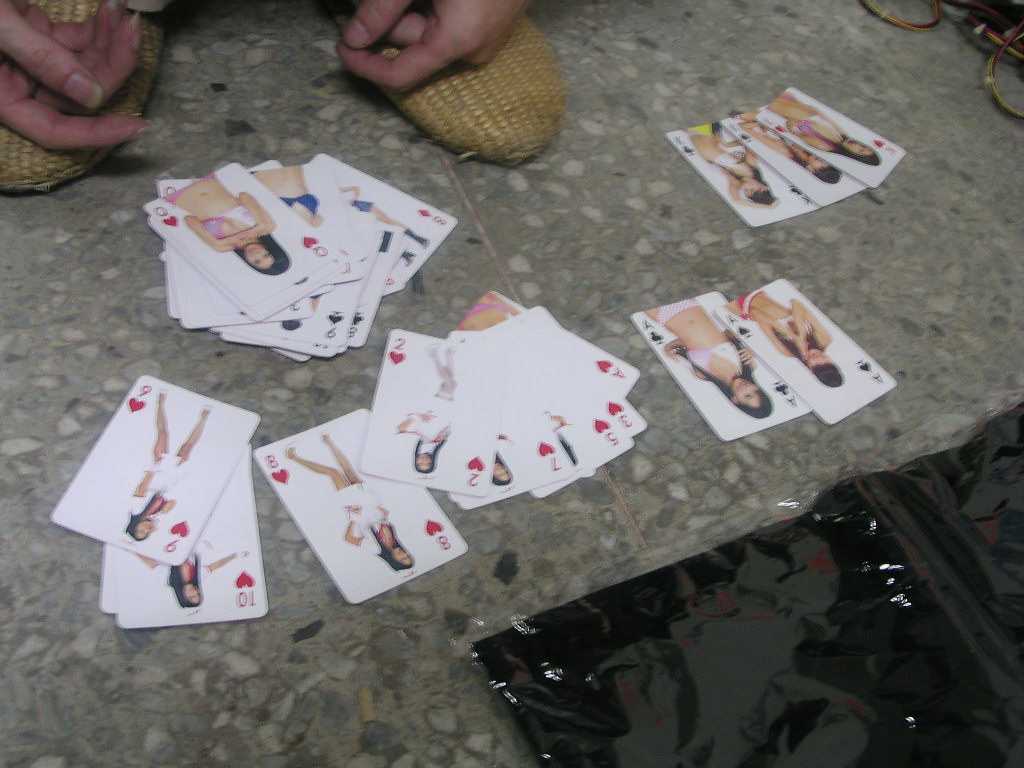A cluttered scene features a rocky tile floor strewn with various playing cards. Each card displays images of actors, particularly women adorned in different outfits. Toward the bottom right corner, some black fragments are visible. On the left side of the image, a person, possibly crouching, extends their hands towards the scattered cards. The top right holds a more organized stack of these playing cards. The overall composition captures the chaotic yet intriguing assortment of themed playing cards on an uneven surface.